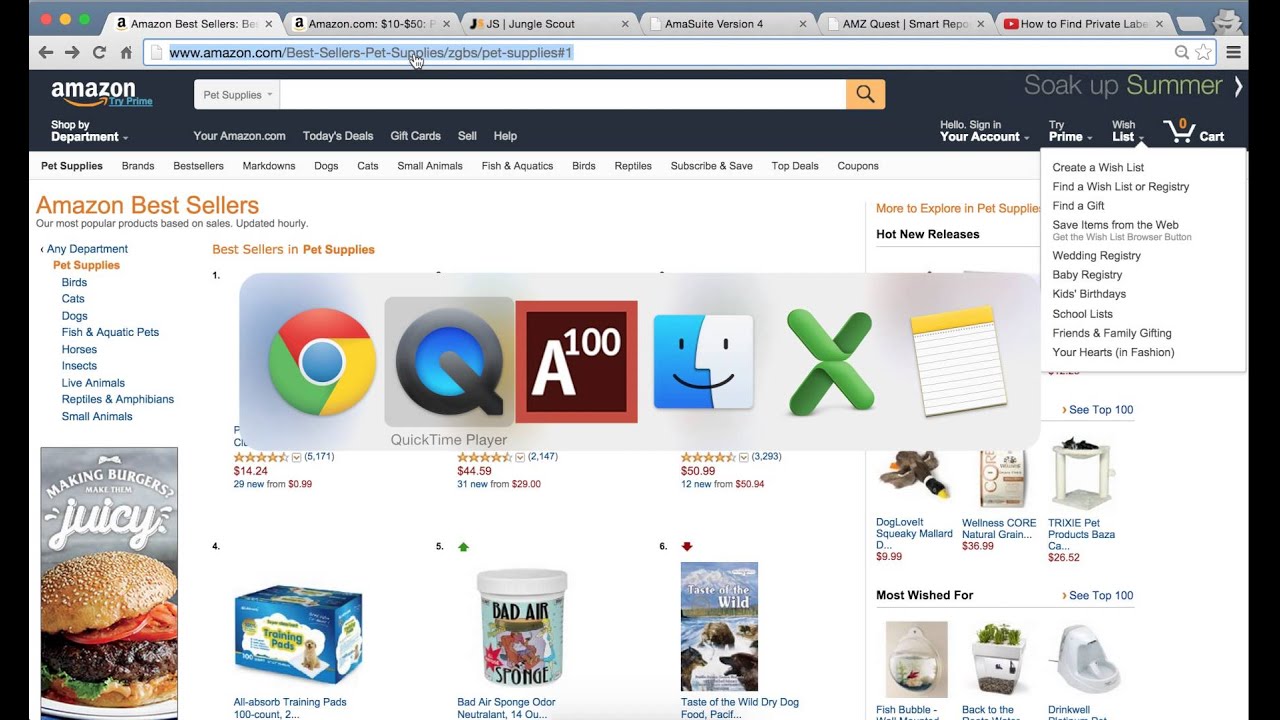The image shows a MacOS interface with Google Chrome open, displaying six browser tabs. The active tab is on an Amazon webpage titled "Amazon Bestsellers" specifically under the "Pet Supplies" category. The visible section of the page features a ranked list of items, although only positions four through six are partially visible due to their small size and the overlay of a task switcher pop-up. The top three items in the list are obscured by this task switcher, which appears to be facilitating quick transitions between Chrome and other applications, such as Notes. The webpage has a predominantly white background, with blue hyperlinks scattered throughout. In the top right corner, there's a section related to wish lists, including options to create a new list, among other functionalities.